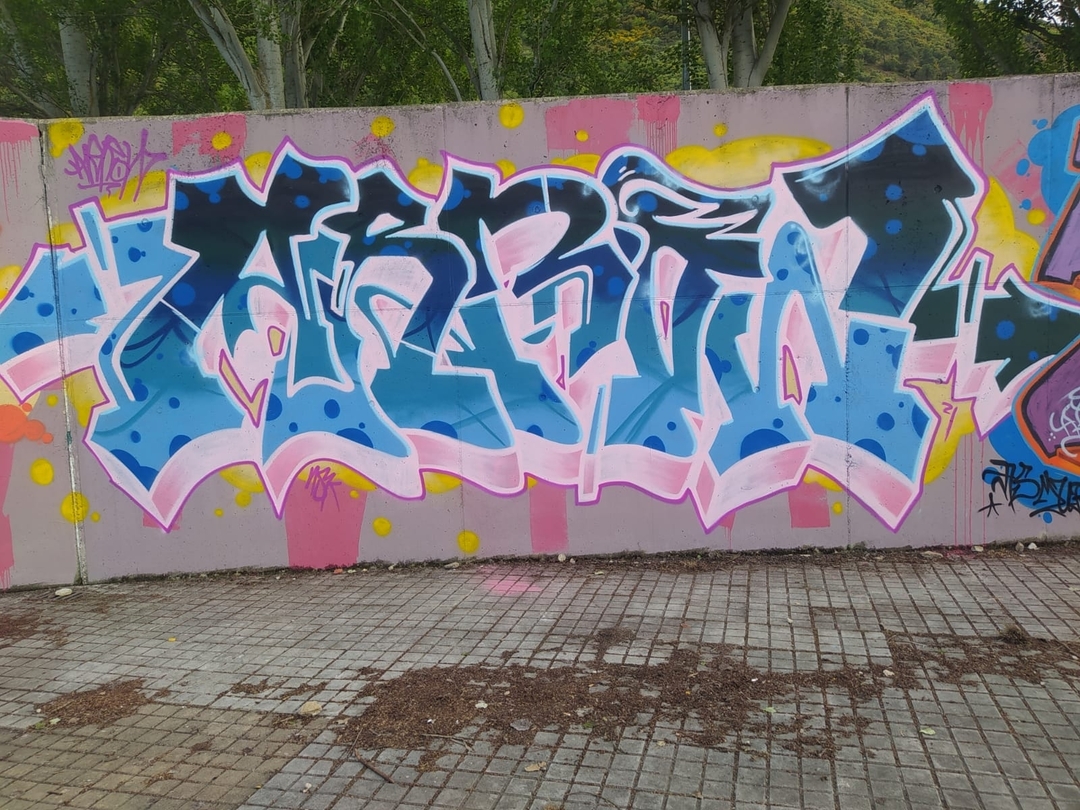The image showcases an extensive graffiti mural on a massive concrete wall that appears gray or lavender, stretching beyond the photograph’s frame. The ground in front of the wall consists of a grid-like pattern of cement tiles interspersed with piles of dirt and debris. A splash of pink paint on the ground hints at some spillage from the mural creation. Rising above the wall, green and slightly yellowing trees contribute to the scene's outdoor and possibly neglected urban environment.

The graffiti itself is an intricate and stylized piece of art, making it almost indecipherable. It seems to spell out "Y-N-P-I-W" in a highly ornamental text. The gradient of colors includes a dark blue at the top transitioning to a lighter blue at the bottom, with blue splotches in the center. Pink outlines and pink and yellow patterns add vibrancy behind the main letters. The entire graffiti has a 3D raised effect, with pink giving the illusion of depth. Additionally, a right-facing arrow in dark blue or green on the right side of the graffiti points towards another piece that features some purple with an orange shadow, though this secondary piece remains largely out of view. The wall also contains some foreign script at the bottom, not in English.

In summary, the photograph vividly captures a colorful and detailed graffiti mural against a backdrop of urban decay, highlighted by dirt-strewn cement tiles and overhanging trees.